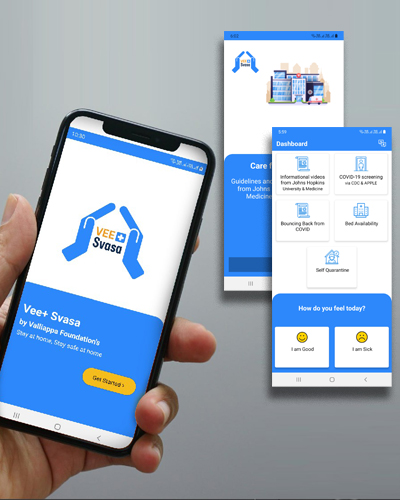In this image, situated in the lower left-hand corner, there is a man's hand, likely belonging to a Caucasian or possibly Asian individual with very pale skin, holding a smartphone towards the camera. The smartphone screen is prominently displayed, with the upper two-thirds showing a white background and the bottom third a beautiful shade of turquoise blue. 

Centrally located on the white background is a logo featuring a simple drawing of two steepled hands, resembling a house. Around this logo is the text "VE" in gold, accompanied by a plus sign enclosed within a blue square. Beneath this, the text "SVASA" is written in a dark blue font. Further down, at the bottom of the screen, we see the same name written again: "VE + SVASA" in a white font against the turquoise background.

In the upper right section of the image, two additional screenshots from the company's website are visible, one slightly overlapping the other. The top of the rightmost screenshot is adorned with the same turquoise blue, labeled as a dashboard. The center area of this screenshot features various icons that, while visible, are too small to decipher. These elements collectively offer an interested viewer a glimpse into the company's digital interface and branding.